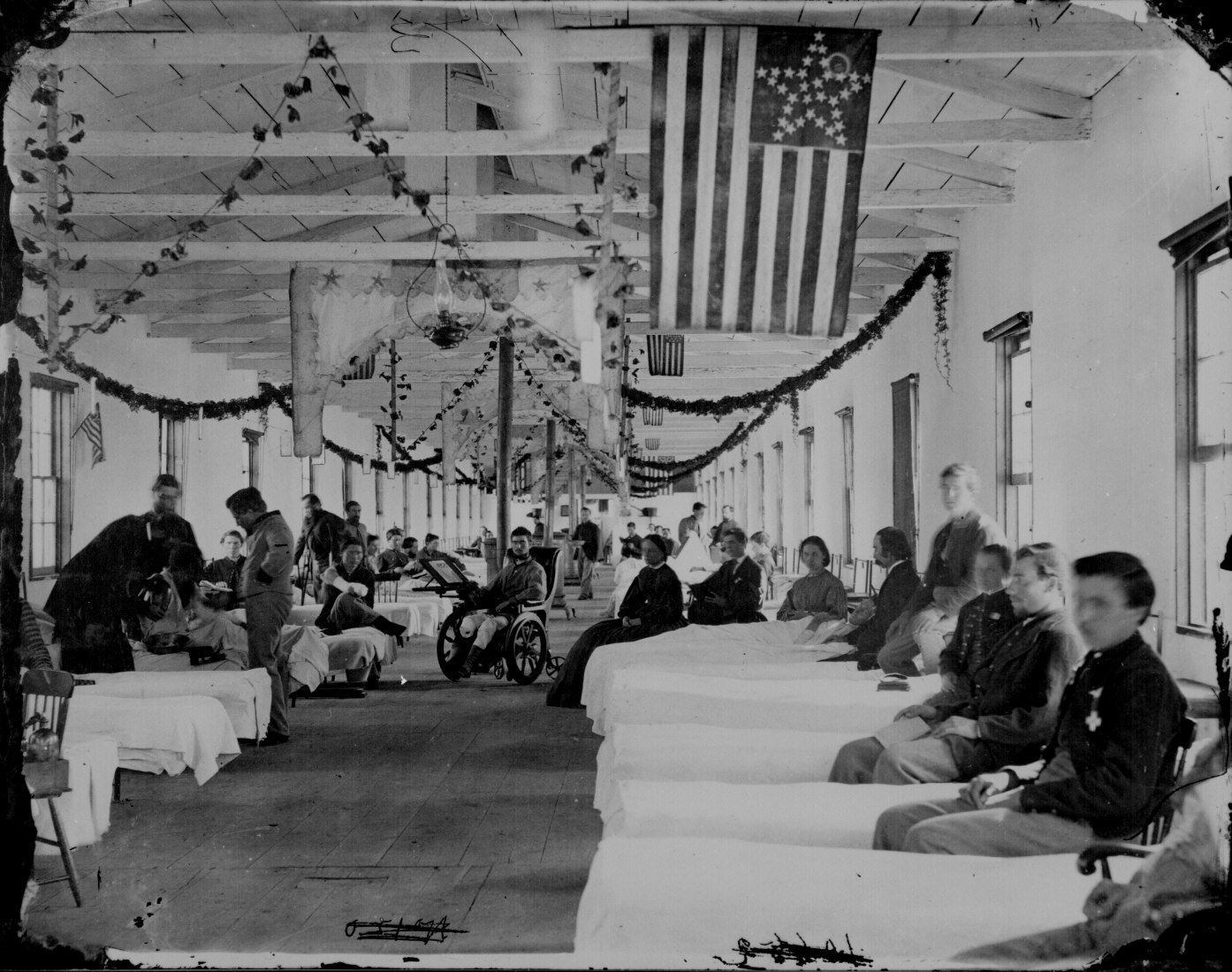This vintage black and white photograph appears to be from a World War I-era military hospital in the United States. The large, open indoor space features rows of hospital beds aligned along both the right and left walls, extending into the distance. Each bed is covered in white linens and is accompanied by a chair, with several men, some in dark shirts adorned with medals and patches, sitting either on or beside the beds. Central to the image is a man in a wheelchair, notably missing one leg, surrounded by people including women sitting nearby.

The hospital room's wooden roof contrasts with its likely plaster or drywall white walls, punctuated regularly by windows spaced about ten feet apart. From the ceiling hangs greenery, perhaps decorative, along with an American flag with an unusual star configuration, where the stars are arranged in a larger star pattern, and there are four stars at the center. Despite some illegible writing at the bottom of the image and signs of significant wear and damage on the edges, the photograph has been carefully scanned to preserve as much visual detail as possible.